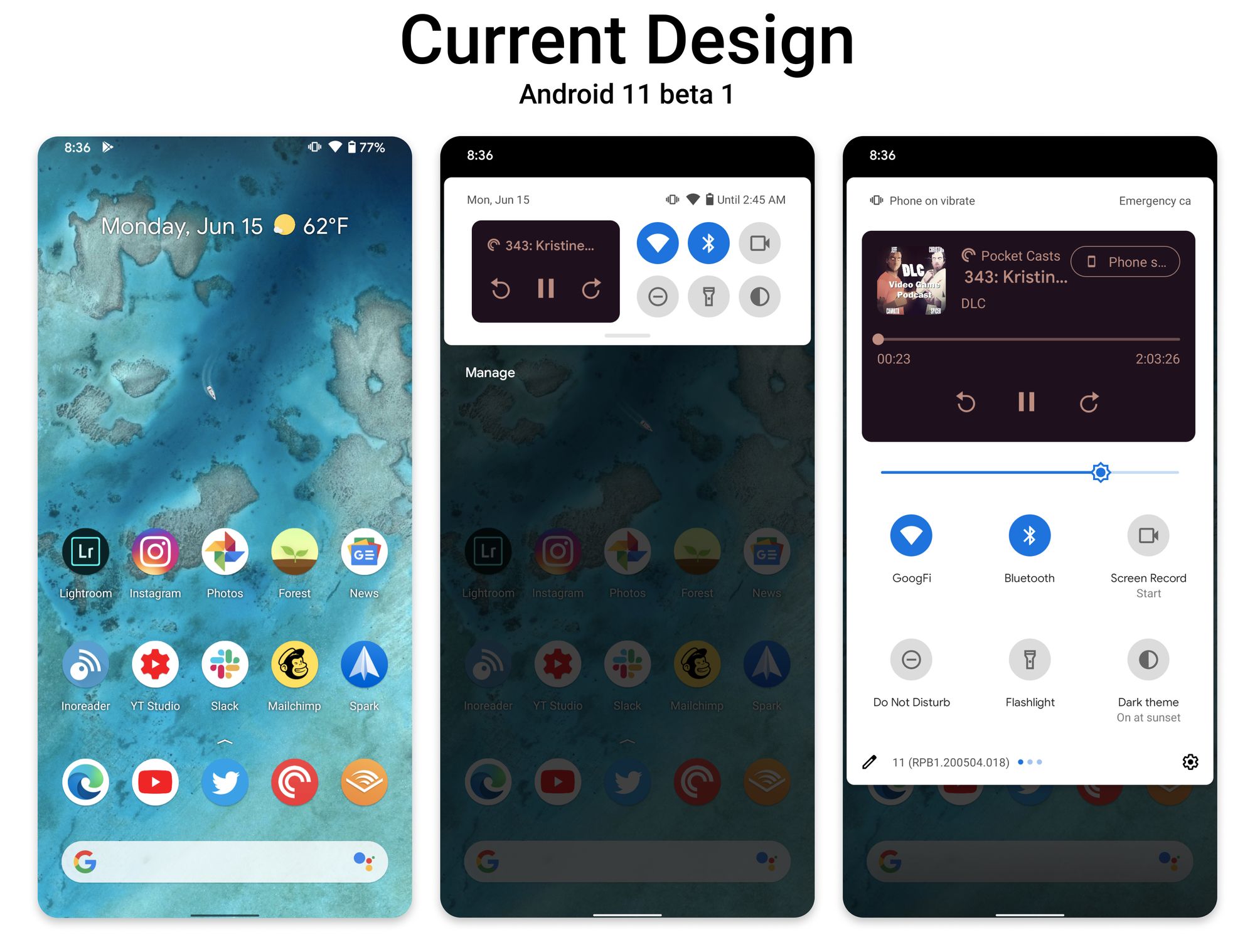**Detailed Caption:**

This image showcases a section labeled "Current Design" on a white background, featuring black text. Directly below that, in smaller text, it reads "Android 11 Beta 1," indicating that the visuals pertain to an early beta version of Android 11, which is now considered outdated.

The image contains three screenshots of the Android 11 interface. The first screenshot, positioned in the upper left, displays a home screen with a purplish-blue background. The top status bar reveals various icons: the time (8:36), a Google Play Store notification, the phone set to vibrate, nearly full Wi-Fi signal strength, and a mostly full battery at 77%. The date indicated is Monday, June 15, with a sunny weather icon and a temperature of 62°F.

Below the status bar, several app icons are visible, including Lightroom, Instagram, Photos, Forest, News, YouTube Studio, Slack, MacUp (text is partially obscured), Spark, Microsoft Edge, YouTube, Twitter, and what appears to be Amazon Booking, though the exact name is unclear. At the bottom of the screen, there is a search bar.

The second and third screenshots feature a pop-up music player interface. The third screenshot, on the far right, includes a larger white background pop-up with black text containing instructions or information relevant to the user. This layout appears to be guiding the user through specific functionalities or settings within the Android 11 interface.